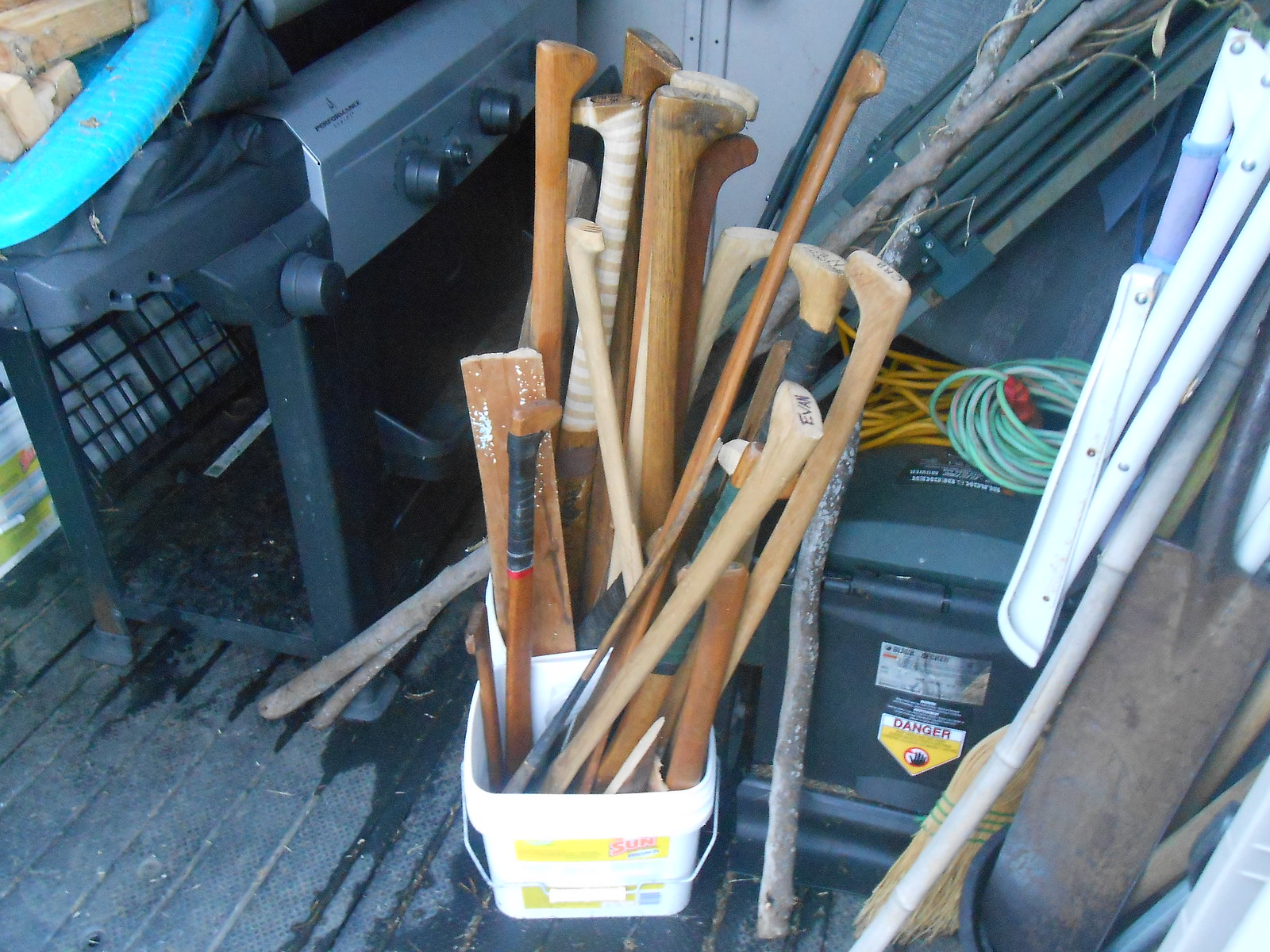The photograph captures a cluttered storage shed with a slightly serrated floor, taken with an older camera. Dominating the center of the image is a white bucket filled with various wooden poles, resembling cane-shaped objects with curved ends. To the left, partially obscured by other items, is a gas grill, identifiable by its silver color, knobs, and two legs, though its propane tank is not attached. Nearby, there is a coiled blue hose and a yellow cord, either for electricity or water, lying atop a box marked with a "danger" sign. On the right side of the image, folded beach chairs hang against the wall, alongside a collection of shovels, including a large brown spade, and a broom. The scene is indicative of a messy storage area or a possible preparation zone for some sort of outdoor gathering.